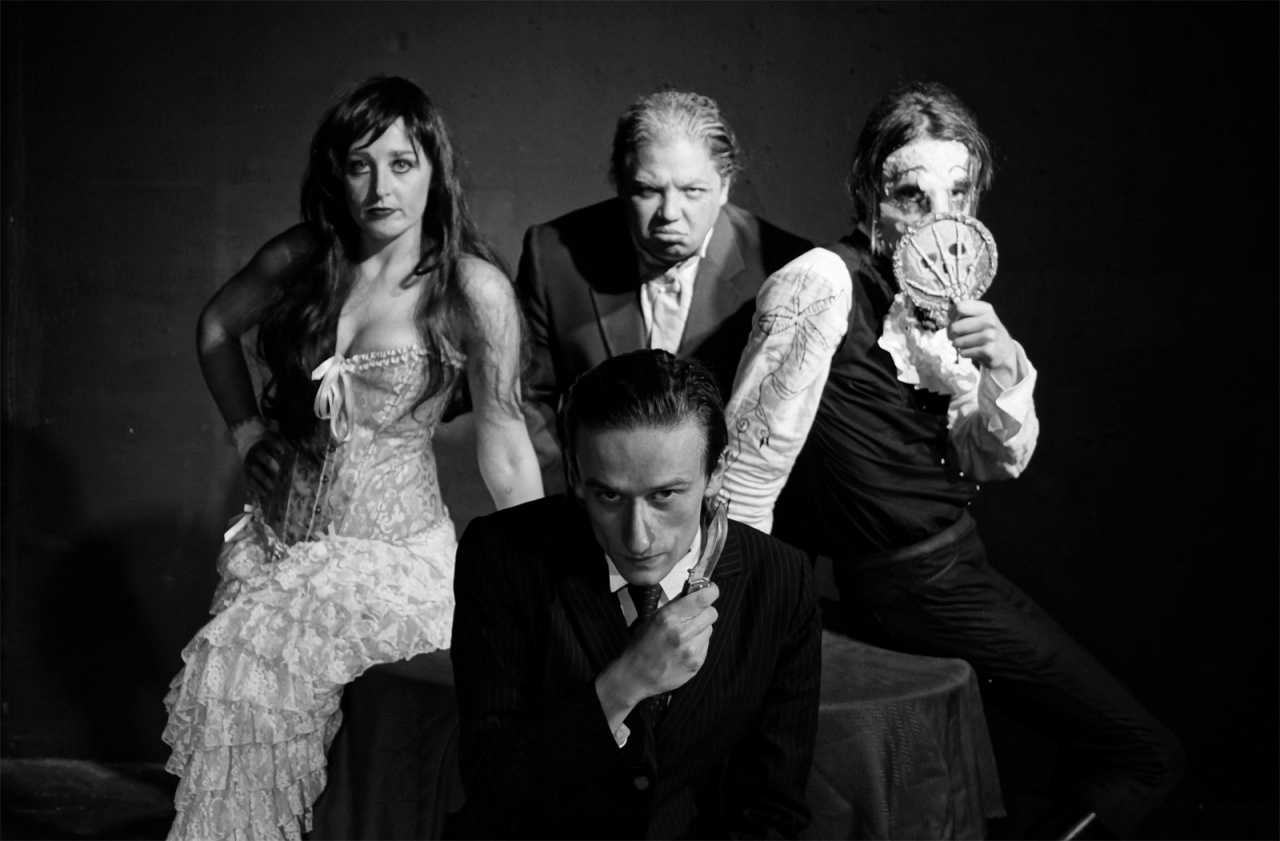In this black-and-white photo, four people are captured exuding an eerie and menacing aura. The foreground is dominated by a man in his 30s with slicked-back dark hair, a longer nose, and an angry expression aimed directly at the camera. Dressed in a black suit and tie, he holds his right hand, which appears to clutch a knife, near his shoulder. 

Behind him, perched on a table draped with a black tablecloth, are three more figures. On the far left is a woman with long dark hair cascading over her shoulders. She dons an elaborate corset and a sleeveless, frilly white lace dress that exposes her arms and slightly reveals her cleavage. To her right stands an older gentleman with graying, thinning hair. He is dressed in a suit with a black jacket, white shirt, and white tie, and he wears a stark, menacing expression. 

The final person, whose gender is difficult to discern, stands next to the older man. This individual has darker hair and is partially masked, covering part of their face with a fan in their left hand. They are attired in a fancy white shirt with frills, a black vest, and black pants or skirt. All four figures appear stern and unwelcoming in this haunting black-and-white composition.